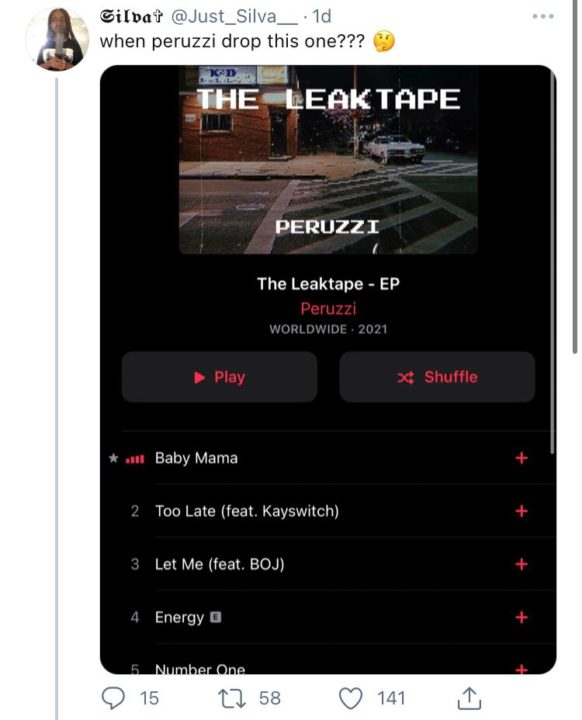A detailed caption for the described image might be:

---

A screenshot of an old Twitter post by a user named "Silla" (@_Silla__). The post, made one day ago, features the tweet: "When Peruzzi dropped this one??? 🤔" along with an image of a music app showcasing Peruzzi's album 'Delete Date'. The album cover displays a dimly lit street at night with a solitary figure crossing, under streetlights. The EP, titled 'Delete Date Dash', released by Peruzzi Worldwide in 2021, lists several tracks: "Baby Mama" (highlighted with currently playing equalizer bars), "Too Late" (ft. K-Switch), "Let Me" (ft. B.O.J.), and "Energy" (marked explicit). Each song is accompanied by a red plus icon, hinting at adding to a playlist or library. The post data includes comments, retweets, and likes, adding to its engagement metrics.

---